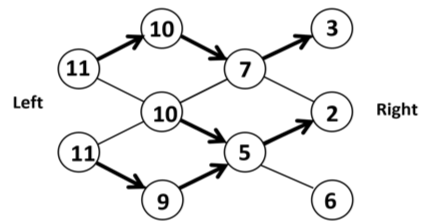Illustration Description: 

The image features a white background with the word "left" in black letters positioned on the left-hand side and the word "right" in black letters on the right-hand side.

On the left-hand side, there are multiple numbers, each enclosed within a circle with a white background and a black border. Arrows connect these circled numbers, depicting a sequential flow:

- An arrow from 11 points to 10.
- 10 points to 7.
- 7 points to 3.
- Additionally, another arrow from 11 points to 9.
- 9 points to 5.
- 5 points to 2.

At the top of the left-hand side, the number 11 appears twice in circles. The first 11 has an arrow pointing to 10, which further points to 7. The second 11 points to a different 10, which in turn points to 5, leading finally to 6.

The overall layout presents a structured diagram with a series of interconnected numbers within black-bordered circles, illustrating two different sequences originating from the number 11.